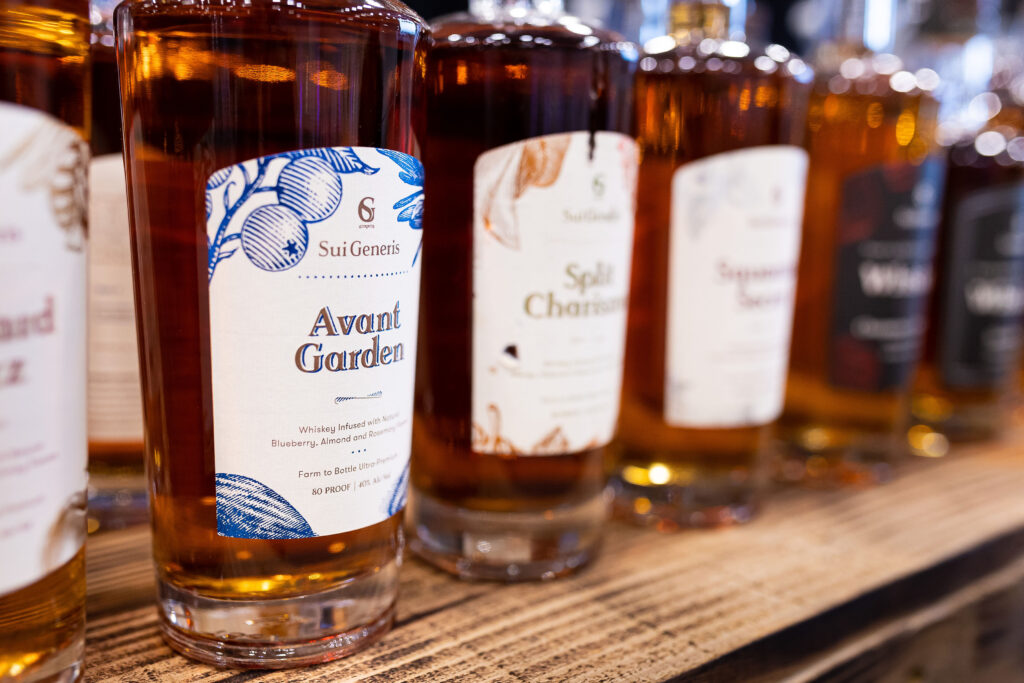The rectangular image, wider than it is tall, features a linear arrangement of several alcohol bottles on a brown stand or bar counter. The most prominent bottle on the left stands out due to its detailed, visible label which reads "Sui Generis of Avant Garden." The label, predominantly white with delicate blue designs that include illustrations resembling blueberries, almonds, and possibly rosemary, conveys it is a whiskey infused with these ingredients. The bottle's label also states "Farmed to Bottle, 80 Proof." The other bottles, with varied designs including brownish and black labels, fade into the background, becoming progressively out of focus towards the right, suggesting a collection of diverse liquors.